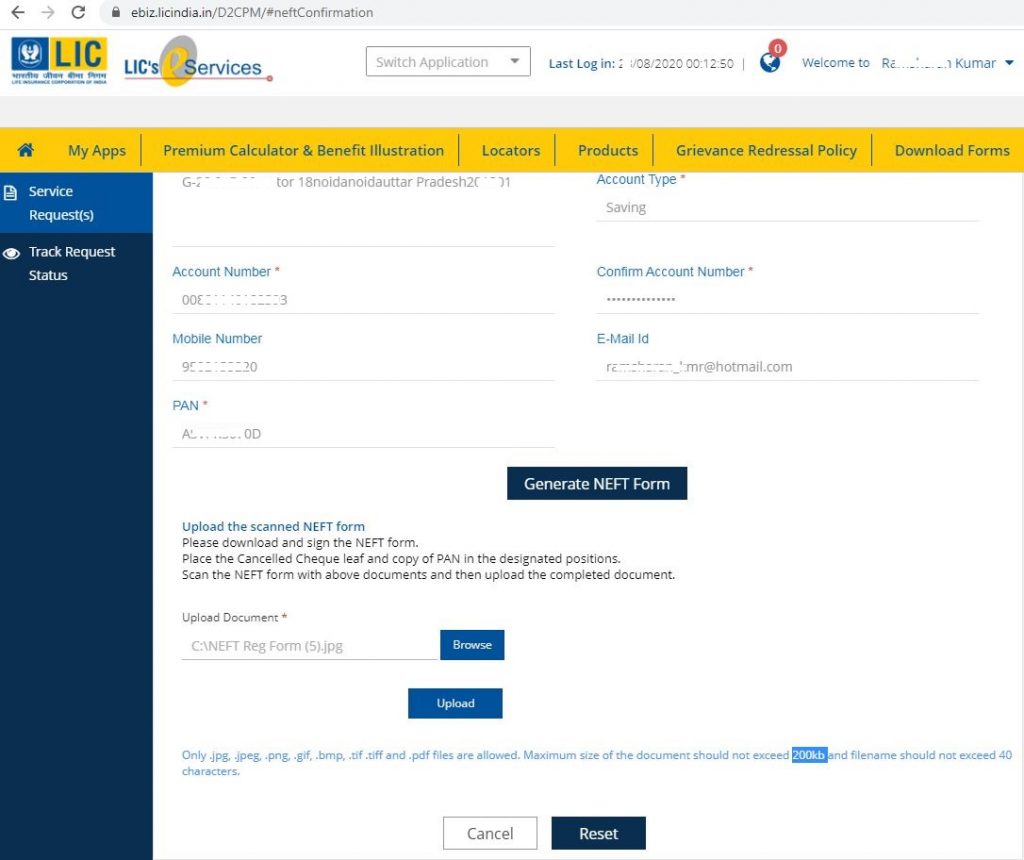The image is a detailed screenshot of a web page, likely viewed on a computer monitor. The background of the web page is predominantly white, with a distinct dark blue column running down the left-hand side, which appears brighter towards the top. Across the very bottom of this blue column is a lighter blue rectangle. At the very top of the screen, there's a light gray bar featuring a padlock icon, indicating a secured web page. The URL displayed reads "ebiz.licindia.in/[rest_of_the_URL]", and to the left of this are a back arrow and a refresh circular arrow.

Below this gray bar is the LIC logo displayed prominently, consisting of large, blue capital letters "LIC" on a yellow rectangular background. Accompanying the logo is a white emblem resembling wings or laurels within a blue square. Next to the logo, it says "LIC's e-Services," where the letter "e" in "e-Services" is noticeably larger and in lowercase yellow compared to the rest of the text, which is blue. 

To the right of this logo setup is a search bar labeled "Search Application." Below it are details like the last login date and time, and an obscured line stating "Welcome to [obliterated] Kumar." 

A yellow menu bar sits underneath this, horizontally listing different clickable options such as "My Apps," "Premium Calculator," "Benefit Illustration," "Locators," "Products," "Grievance Redressal," "Policy & Download Forms."

In the blue column on the left, two sections titled "Service Requested" and "Track Request Status" are visible. "Service Requested" seems to be currently highlighted, indicated by its lighter blue color. This section contains a white form with blue headings. The form fields include a blue-labeled "Confirm Account Number," with the actual account number obscured by dots or asterisks. Below are details like "Account Type," marked as "Saving." 

At the bottom of the form, there is a button labeled "Generate eNFT Form." This page also features options such as "Cancel" and "Reset" at the very bottom, hinting at functionality possibly related to government benefits or another formal service.